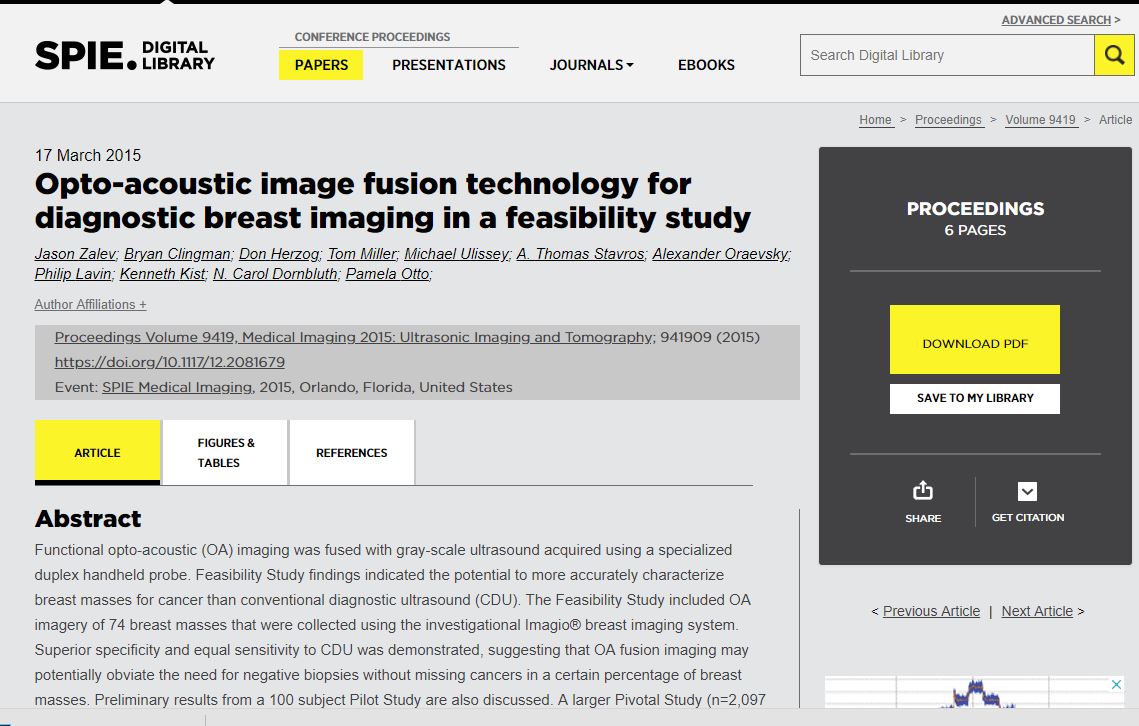This image features the homepage of the SPIE Digital Library, a searchable digital repository prominently known for its gray-themed interface accented with black and yellow highlights. These color elements evoke a similarity to the Pittsburgh Steelers' color scheme. At the top-left corner of the screen, the title "SPIE Digital Library" is displayed in bold, immediately capturing the user's attention. 

Adjacent to the title, there are several interactive drop-down menus labeled "Conference Proceedings," "Papers," "Presentations," "Journals," and "E-books," providing quick access to various types of content available within the library. To the right of these menus, a search box is situated, allowing users to conduct general searches or utilize the advanced search feature for more specific inquiries.

Beneath these navigational elements, the primary section of the webpage displays an array of medical journals and articles, indicating the library's extensive collection of medical literature. Users are offered functionalities such as downloading articles in PDF format and organizing selected items into a personalized library. The organized layout and user-friendly features of the SPIE Digital Library facilitate efficient access to a wealth of scholarly resources.